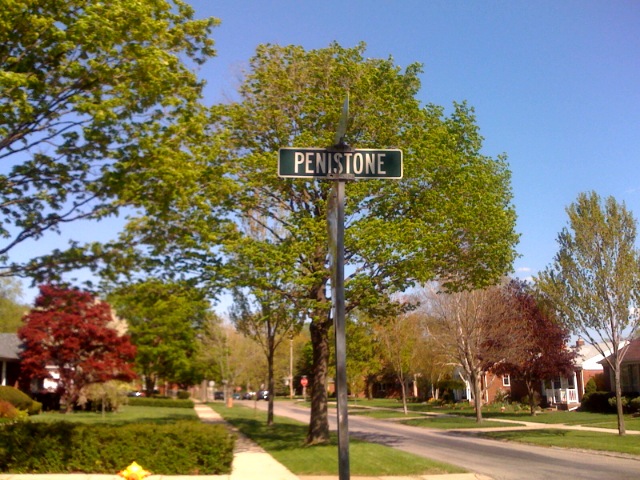This landscape-oriented colour photograph captures a typical suburban street in the United States during daytime. In the foreground, a classic American street sign stands out, supported by a grey metal pole. The prominent horizontal sign displays the name "Pennistone" in white text against a dark green background. Just above it, another green and white street sign is visible from the side, but its text is obscured. The scene includes a standard North American road flanked by green verges, sidewalks, and front gardens with neatly trimmed hedgerows on both sides. Large trees with varied foliage - some green, some brown, and others with red leaves - line the streets, partially veiling the houses. A colorful mix of a burgundy tree on the right and light green trees on the left enhance the picturesque suburban setting. The clear, brilliant blue sky overhead completes this tranquil neighborhood scene.